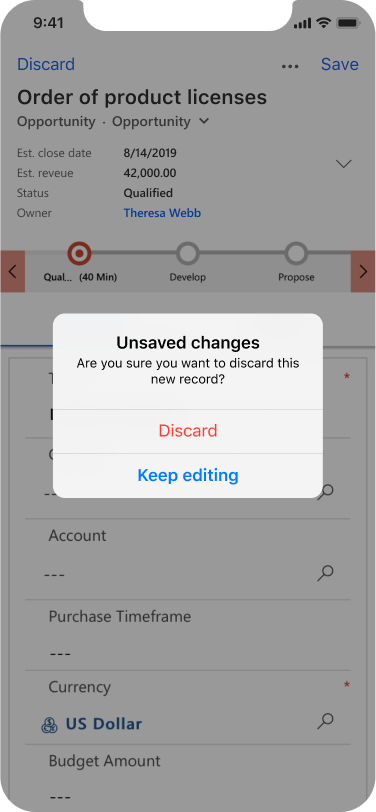The image depicts an iPhone screen divided into two main sections. In the background, there is an order page for product licenses, highlighting several important details. The page lists an estimated close date of April 14, 2019, with an anticipated revenue of $42,000. The order is currently marked as 'qualified' and is owned by Teresa Webb. Various settings such as currency, budget amount, and purchase time frame are also visible, suggesting a complex, business-to-business transaction.

In the foreground, a pop-up dialog has appeared, asking the user to confirm if they want to discard a new record. The dialog gives two options: 'Discard' in red font or 'Keep Editing' in blue font. From the interface elements, it is apparent that the device in use is an iPhone. This confirmation window hints that the user may have accidentally or intentionally clicked on a setting to delete or discard the action, possibly affecting the order shown in the background. The image captures a moment of decision, indicating the critical nature of managing business transactions accurately.